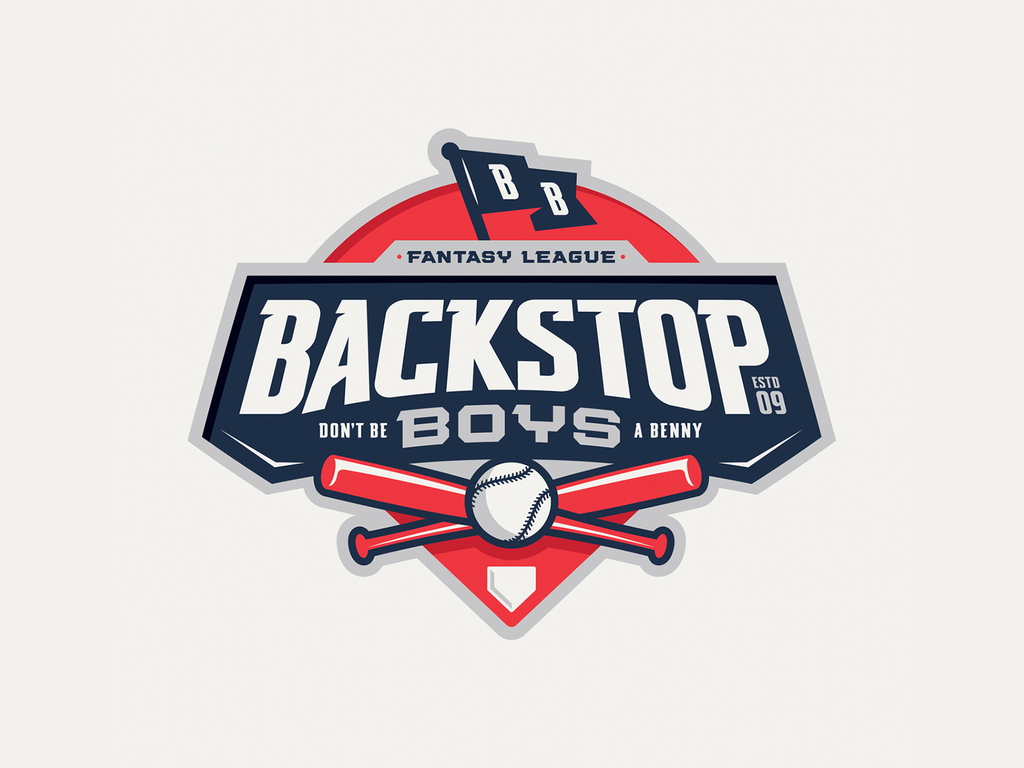This colorful logo, set against a light gray or off-white background, represents a fantasy baseball league. The design features a large, dark blue pennant at the top, emblazoned with "BB" in white lettering, indicating "Backstop Boys". Below the pennant, the words "Fantasy League" are prominently displayed in a dark blue font. The central focus is the team's name, "Backstop Boys", written in bold white letters, surrounded by the phrase "Don't Be a Benny". Below this, in a blue and white color scheme, the text "established 09" is visible.

The lower part of the logo incorporates elements of a baseball diamond, highlighted in red, showcasing the white home plate. Dominating this section is a large white baseball with blue stitching, centrally placed over two crossed reddish-orange bats. The intricate details and the mix of colors — dark blue, orange, white, and grey trim — provide a dynamic and eye-catching emblem for the Backstop Boys fantasy baseball league.